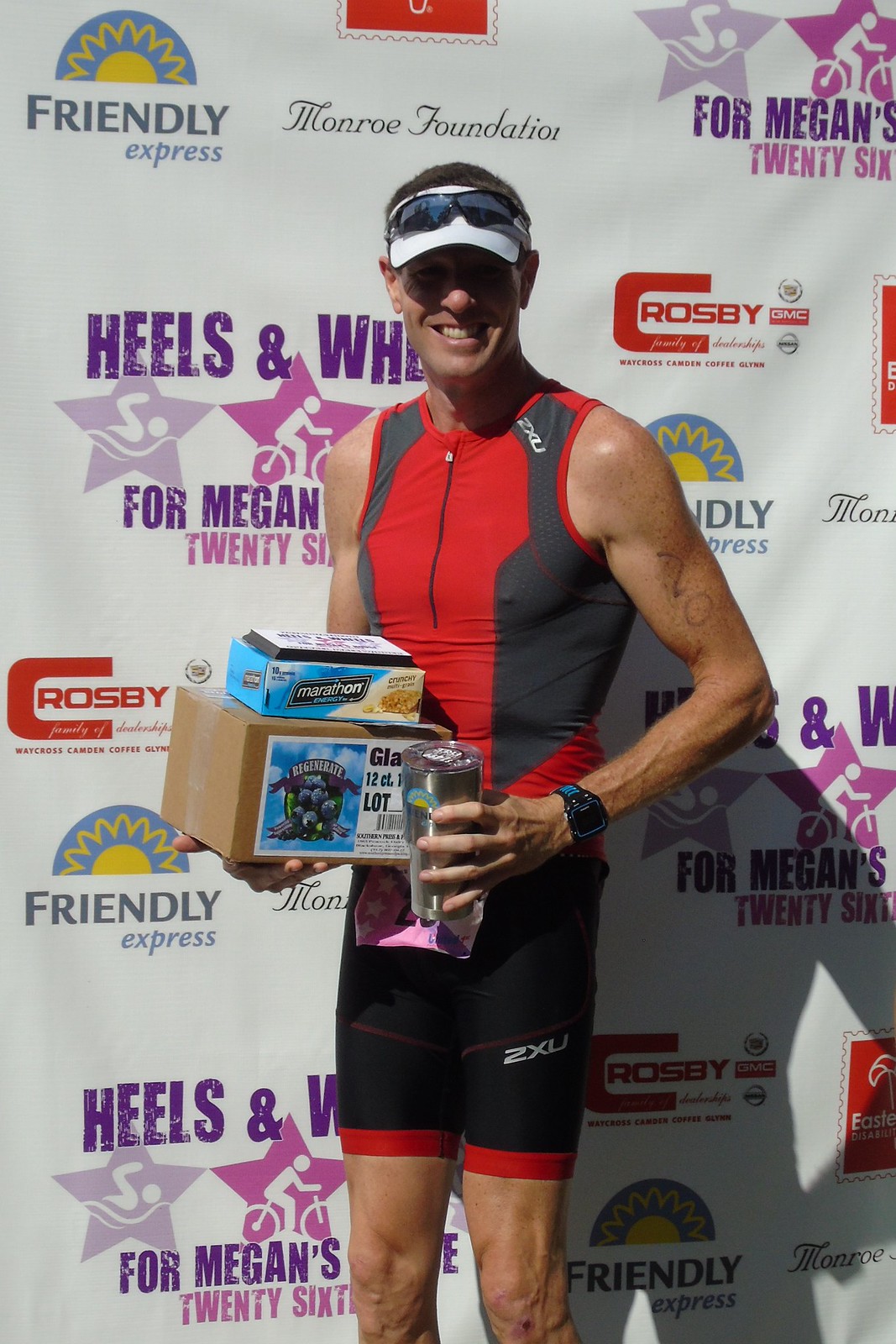The photograph captures an athletic-looking man standing outside, discernable from the lighting conditions. He's positioned in front of a white banner adorned with various logos, including Friendly Express, Monroe Foundation, Crosby GMC, and Heels and Wheels for Megan's 26th, among others. The man is dressed in cycling attire, featuring a tight, sleeveless red and dark gray top with a half-zip front and black bicycle shorts with red trim at the bottom. He sports a white visor with sunglasses resting atop it and a smartwatch on his left wrist. In his right hand, he holds a stack of two boxes: a cardboard box labeled "GLA 12-count lot" and, on top of it, a blue and white box that reads "marathon" and possibly contains crunchy bars with some papers or a smaller box on top. His left hand grips a silver metal tumbler with a plastic lid and the Friendly Express logo on it. The man is smiling, suggesting a sense of accomplishment or joy, likely related to the event noted on the banner behind him.